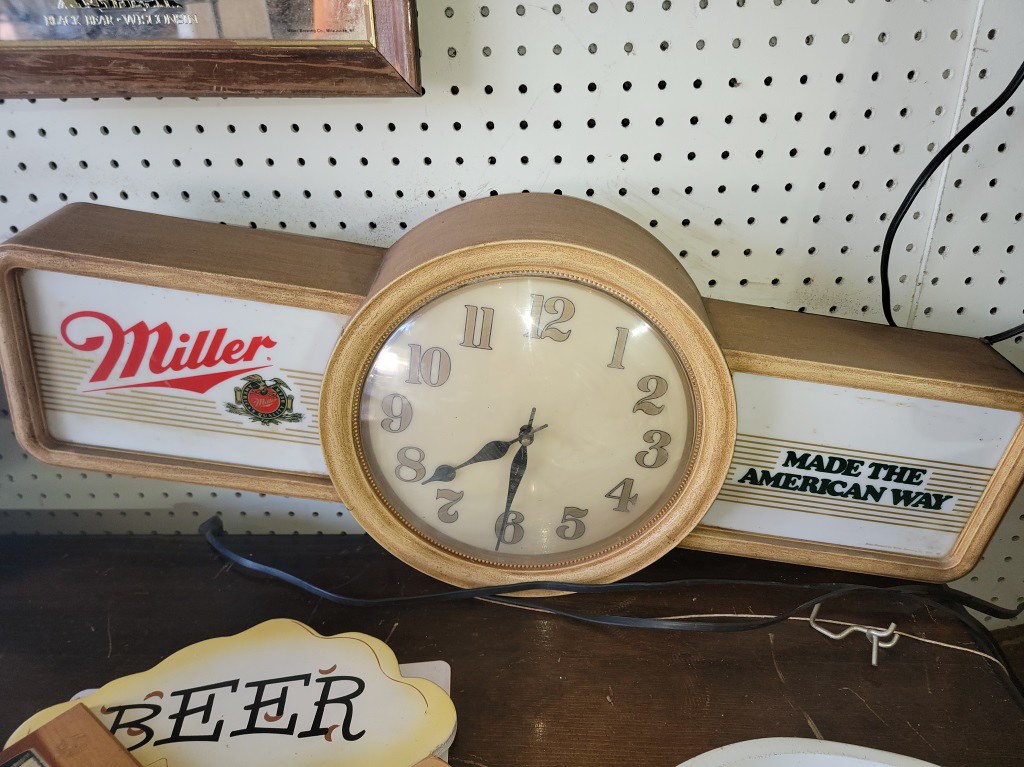The image depicts a vintage, rectangular wall clock prominently featuring a beer logo. The clock is long, thick, and made primarily of wood, with certain elements encased in white plastic. At the top center of the clock is a round clock face with a tan background and golden numbers outlined in black.

On the left side of the clock face, the iconic Miller logo is displayed in bold red letters, angled to the right, with gold stripes beneath the logo. The right side of the clock features a white background with gold stripes, and within these stripes, the phrase "Made the American Way" is written in thick black letters.

The clock is positioned at an angle on a brown desk, with the left side elevated and the right side resting on the desk, causing the Miller logo to tilt upwards. There is a visible black power cord wrapped around the desk, which is notably scratched and worn. In the top left corner of the photo, part of a wooden frame can be seen, while the bottom left corner shows the top of a sign with the word "beer" in large black letters.